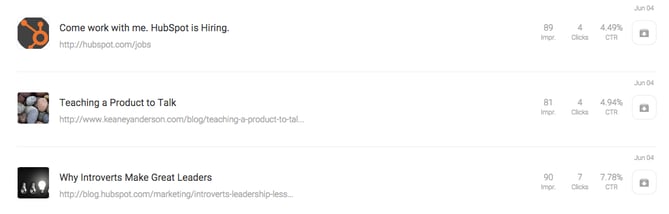The image is a screenshot of an analytics page, with a clean, white background and minimal content. The page appears to be either a social media analytics dashboard or a blog/article performance overview. The layout features three entries, each spanning a single line with a small photo on the left, followed by the name of the blog or article, the web address, and various engagement metrics to the right.

1. **First Entry:**
   - **Photo:** A logo or promotional image.
   - **Title:** "Come Work with Me, HubSpot is Hiring."
   - **Web Address:** Displayed beneath the title.
   - **Metrics:** 
     - Impressions: 89
     - Clicks: 4
     - Click-Through Rate (CTR): 4.49%
     - Date: June 4th

2. **Second Entry:**
   - **Photo:** A stock image, close-up of pebbles.
   - **Title:** "Teacher, the Product, the Talk."
   - **Web Address:** Displayed beneath the title.
   - **Metrics:** 
     - Impressions: 81
     - Clicks: [not fully visible or unspecified]
     - Click-Through Rate (CTR): [not fully visible or unspecified]
     - Date: [not fully visible or unspecified]

3. **Third Entry:**
   - **Photo:** Another generic stock image.
   - **Title:** "Why Introverts Make Great Readers."
   - **Web Address:** Displayed beneath the title.
   - **Metrics:** 
     - Impressions: [not fully visible or unspecified]
     - Clicks: [not fully visible or unspecified]
     - Click-Through Rate (CTR): [not fully visible or unspecified]
     - Date: [not fully visible or unspecified]

The screenshot captures basic performance data such as impressions, clicks, CTR, and the publication dates for each entry, constructed in a straightforward manner.